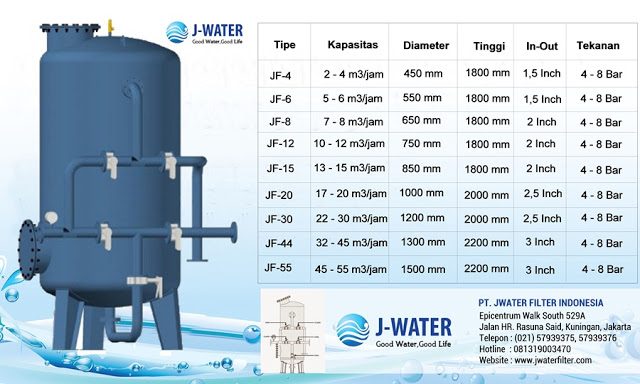The image showcases a detailed specification chart for a water filtration system by Jay Water Filter Indonesia. On the left side is a blue 3D illustration of the water filter, complete with multiple pipes and a representation of water and bubbles beneath it. Above the filter is the company's logo—a sphere with white ripples—accompanied by their slogan, "Good Water, Good Life." The right two-thirds of the image contain various specifications including type, capacity, diameter, and length. These are listed in what appears to be Indonesian, with measurements primarily in the metric system, except for the in-out dimensions, which are in inches. The term "tekanan" is noted, with measurements in bar. Additional text includes the company's name, PT Jay Water Filter Indonesia, and their website, www.jaywaterfilter.com.